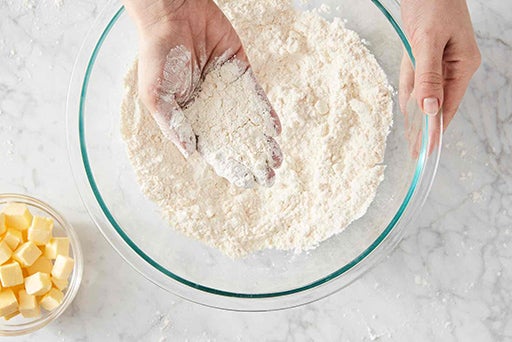The image is a detailed photograph capturing a baking scene from an overhead perspective. At the center of the image lies a transparent glass bowl filled with clumpy white or cream-colored flour, outlined by a thin green border. To the right, a woman's right hand is grasping the edge of the bowl, steadying it on a white surface with a gray marbled design. Her left hand, positioned above the bowl, is palm side up and covered in a dusting of flour. In the bottom left corner of the image, there's another smaller glass bowl containing neatly cubed yellow butter. The entire scene is set indoors, likely in a kitchen, and incorporates a range of colors including white, beige, turquoise, green, yellow, and gray.